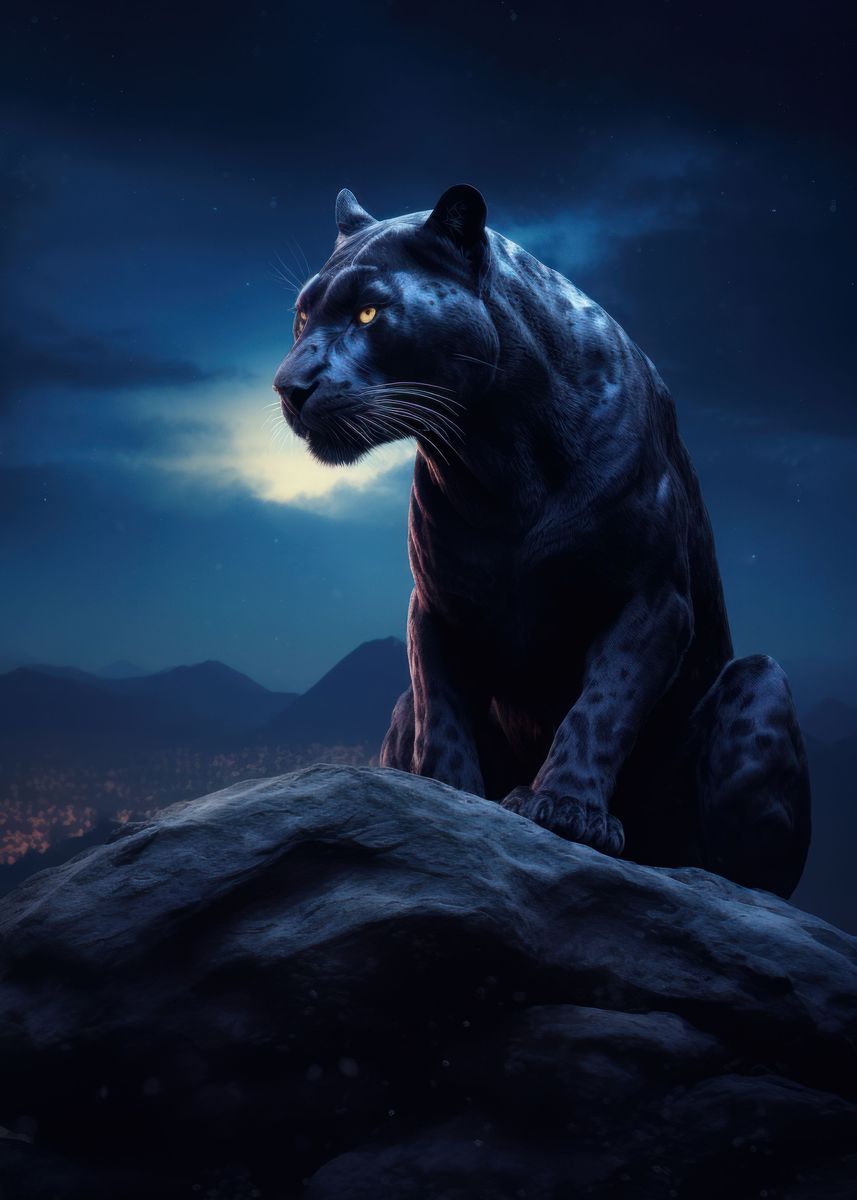In this detailed, stylistic, computer-generated drawing of a fantastical outdoor setting, a black panther with striking light yellow eyes and white whiskers dominates the scene. The panther, with its sleek body adorned with faint black spots, stands majestically atop a dark boulder, central but slightly to the right of the image. The creature appears to have subtle hints of light gray and blue shading on its form, adding depth to its otherwise dark figure. It gazes intently to the left, exuding an aura of mystique.

The background is a dark, enchanting night sky, with deep hues of navy and teal spreading across it. A bright celestial body, possibly the moon or a setting sun, casts a faint glow, giving the scene an otherworldly feel. This celestial light reflects gently off the back of the panther, highlighting its contours. 

In the distance behind the panther, shadowy mountains rise, and below them, faint, blurry lights suggest the presence of a distant city. This fantastical landscape, with its cosmic and mystical ambiance, is artistically rendered within a rectangular frame, evoking the sense of a mythical realm.